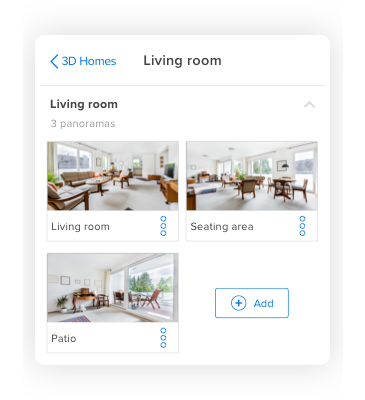The image displays the detailed layout of a home's living room in a 3D panorama format. At the top left of the page, the text reads "3D Homes," with "Living Room" prominently featured across the upper section. The page showcases three distinct pictures, each offering a unique perspective of the living room.

1. The first image, located on the left, captures the spacious living room adorned with white carpet, walls, and ceiling. Despite the blurriness, the large room's expanse is noticeable, taken from one end to encompass as much area as possible. Below this image, the label reads "Living Room."

2. The second picture, positioned to the right of the first, presents a different angle of the same living room, focusing more on the seating area. This shot highlights a couple of tables accompanied by chairs arranged around them. The label "Seating Area" beneath the photo identifies its primary focus.

3. The third and final image, situated below the first two, provides a view near the outside window. The label "Patio" suggests an inside-out perspective, showing part of the interior alongside the exterior patio. Visible in the room are a table leaning against the wall, a plant, and a chair, while the patio outside features additional chairs.

Together, these pictures offer a comprehensive visual tour of the living room, capturing its various sections and furnishing details.